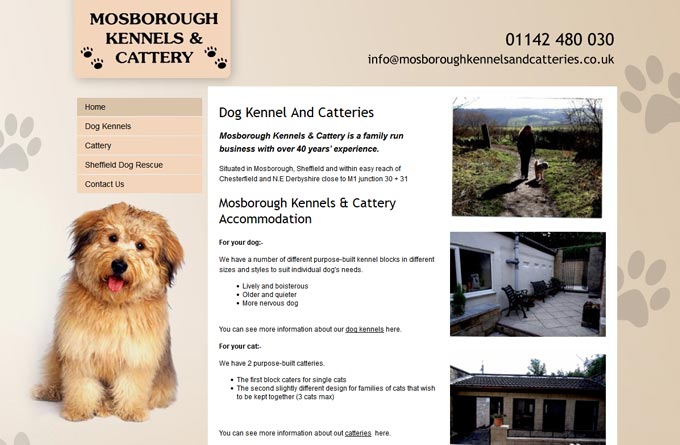The image features a promotional banner for "Mossboro Kennels & Cattery." The entire background is a gradient of beige, starting lighter on the left and darkening towards the right. At the top, in prominent text, the banner reads "Mossboro Kennels" followed by "Cattery." Accompanying the text are paw prints, which add a playful touch to the design.

Taking center stage is a photograph of an adorable, fluffy, brownish-tan dog with long hair, looking directly at the camera with its tongue playfully sticking out. Above the dog, a navigation menu lists options for "Home," "Dog Kennels," "Cattery," "Sheffield Dog Rescue," and "Contact Us."

Toward the top, a contact phone number and the email address "info@mossborokennelsandcatterys.co.uk" are clearly displayed. Below the dog, there's detailed text about the services offered by Mossboro Kennels and Cattery. It mentions accommodations for different types of dogs—lively and boisterous, older and quieter, or more nervous—highlighting the availability of various purpose-built kennels in different sizes and styles to suit individual needs.

On the right side of the banner, there are three pictures showcasing the different kennel accommodations available, providing a visual insight into the facilities offered by Mossboro Kennels and Cattery.